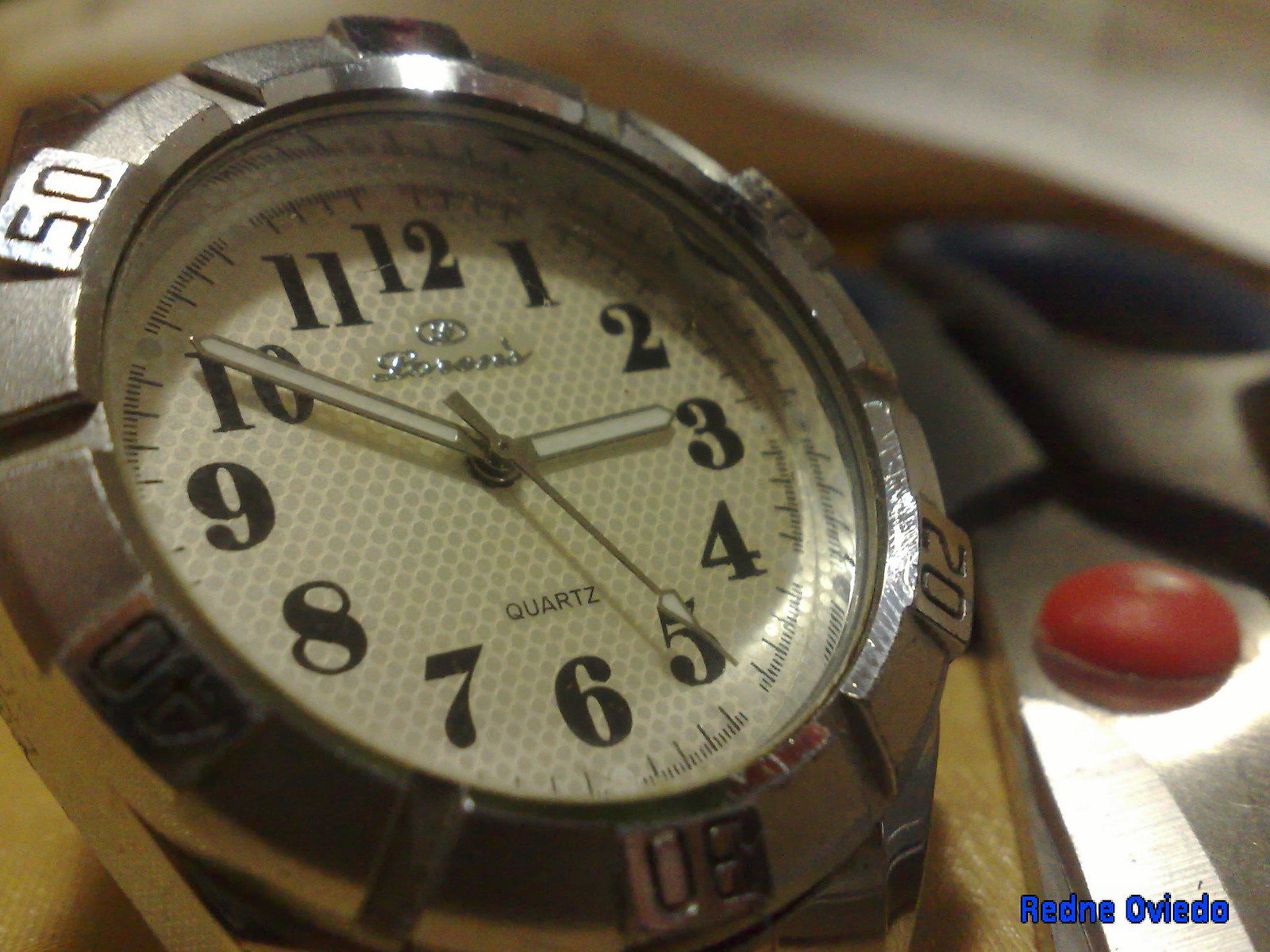This close-up image depicts a robust diver's watch, characterized by a white honeycomb-patterned face that subtly blends in from afar. Under the 12 o'clock position, there's a cursive brand name, possibly 'Larson’s' or 'Boren’s,' accompanied by an oval logo with indistinguishable details. The watch face prominently displays black Arabic numerals in a New Times Roman style, and the word "Quartz" is visible below the center.

Each number, marked every 10 seconds (10, 20, 30, 40, 50), encircles the perimeter, indicating its use for precise timekeeping likely crucial for divers or aviators. The hands are primarily silver with white inlays, though the second hand is entirely silver with a white tip, currently pointing at the 25-second mark.

The watch also features a red button on the right side and an indecipherable phrase, "REDNE OVIEDO," in the bottom right corner. Its solid metal outline and additional intricate markers further underscore its detailed craftsmanship.